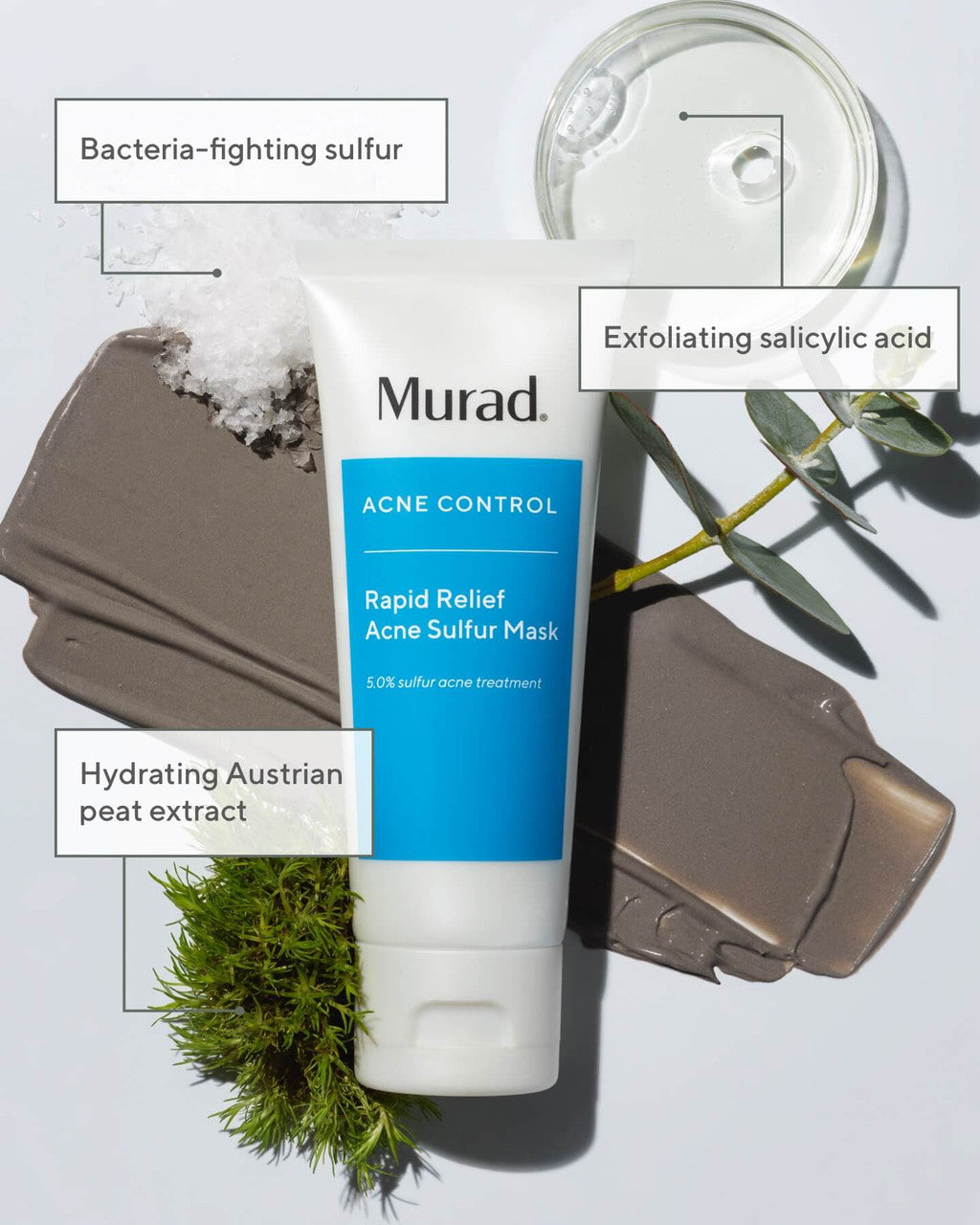The image features a top-angle view of a digital advertisement showcasing a squeezable container of Murad Acne Control Rapid Relief Acne Sulfur Mask, with "ACNE CONTROL" prominently displayed in white, capital letters on a bright white label. The product, a white tube with a white cap, is placed on a light gray surface next to a brown leather pouch. Key ingredients are annotated in white rectangles: "Bacteria Fighting Sulfur" beside some white salt, "Exfoliating Salicylic Acid" near a small glass bowl containing liquid, and "Hydrating Austrian Peat Extract" adjacent to a green plant with leaves at the bottom left corner. A clear petri dish is also present in the top right side of the image, enhancing the scientific aspect of the product’s presentation.